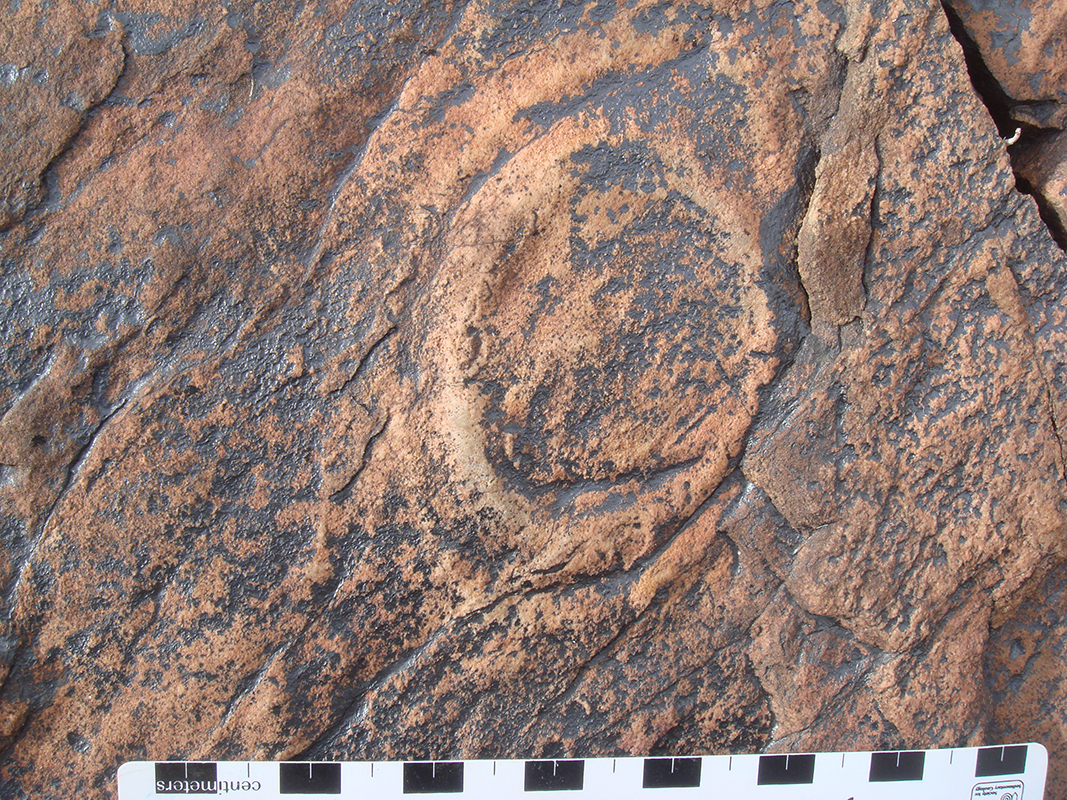This is a detailed color photograph taken outdoors during the daytime, capturing an up-close section of a large rock or the side of a mountain. The rock predominantly displays a light clay-like brown color interspersed with black specks and lines that extend vertically and diagonally across its surface, creating natural ridges and crevices. In the center of the rock, there is a noticeably lighter, rounder spot. At the bottom of the image, a black and white ruler, marked in centimeters, spans almost the entire width of the photo. The markings, which alternate between black and white, are clear and distinct, though the text on the left side is upside down. The overall scene focuses entirely on the rock and the ruler, with no other text or people present in the image.